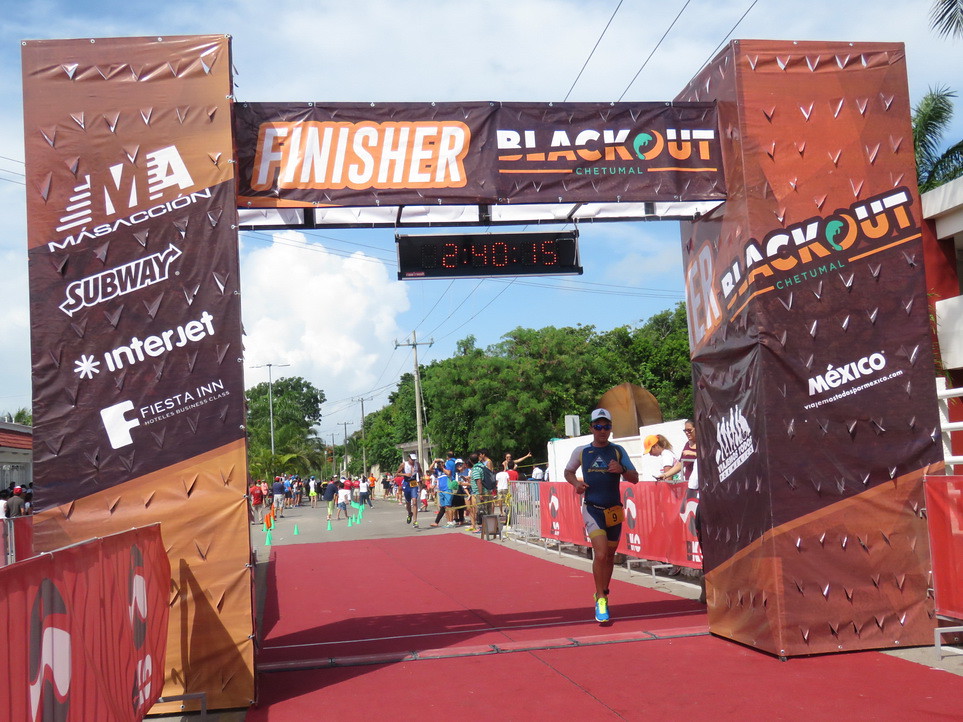In this vibrant, outdoor scene, the photograph captures the finish line of a marathon-style race. Dominating the foreground is a tall archway, flanked by large brown podiums, which spans across the end of the course, about 20 feet above the ground. The archway bears multiple sponsor logos including Subway, Interjet, and Fiesta Inn. Prominently displayed across the top is a banner reading "Finisher Blackout Chetumal." Suspended from the archway is a digital timer, currently showing 2 hours, 40 minutes, and 15 seconds.

The final 25 yards of the race are lined with a striking red carpet, guiding runners toward the archway. Racer number 9, a man appearing to be in his 30s, dressed in a blue top, white shorts with yellow trim, blue tennis shoes, and a baseball hat, is captured just as he crosses the finish line. Encircling the red carpet are blue-green cones delineating the course, and surrounding these boundaries are numerous spectators. Around 40 to 60 people are gathered, some eagerly watching and others capturing the moment with their cameras.

The backdrop reveals an urban setting with a blend of lush green trees and a small brick building to the left. Telephone wires stretch along the road, adding an urban touch to the scene. Above, a beautiful blue sky dotted with puffy white clouds bathes the city in bright, warm sunlight, adding to the celebratory atmosphere of the race finish.